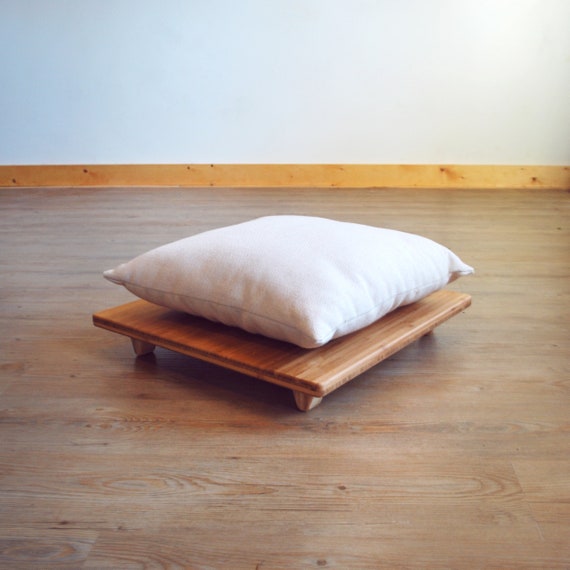In the center of the image, there is a small square wooden platform with short, sturdy legs, approximately one or two inches tall. The platform is brown and features distinct lines that exhibit various shades of brown, enhancing its texture. Atop this platform sits a white, square pillow, with visible stitching along its sides. The pillow appears crisp and clean, contrasting with the wooden tones beneath it. The setting includes a hardwood floor, also brown, that complements the platform. In the background, we see a grey wall meeting the floor, delineated by a baseboard. The light source seems to come from the top right, casting subtle shadows that add depth to the scene.